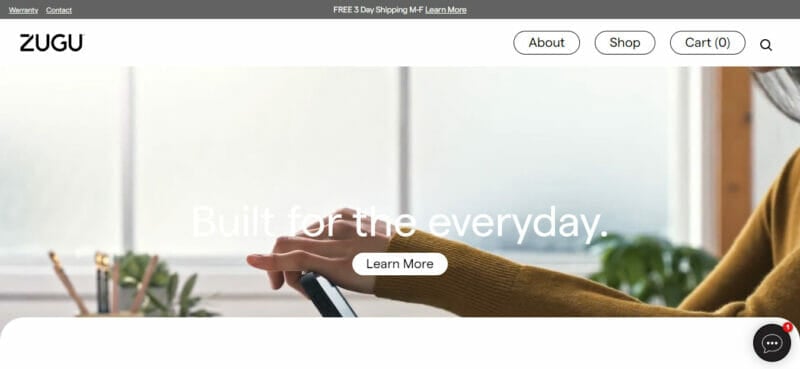The image is a detailed screenshot of the homepage of a website called Zoogoo (or ZUGU). At the very top, there is a gray bar featuring warranty and contact links on the left, and a centrally located notice proclaiming "Free three-day shipping, Monday to Friday" abbreviated as "M to F" with a "Learn More" link. Beneath it, a white bar hosts the Zoogoo logo on the left, while on the right, there are navigation buttons labeled About, Shop, and Cart (the latter being currently empty), along with a magnifying glass icon for search functionality.

Located below these bars is a prominent main image, which showcases a bright and sunny office setting with large windows and visible plants in the background. The image, slightly blurred, captures a person's hands and partial torso, suggesting they are working at a desk with a laptop. Notably, the person is wearing a gold sweater. Overlaying this image is the text "Built for the Everyday" in white font, with a "Learn More" button positioned beneath it. At the bottom right of the page, there's a button represented by a chat bubble, likely for customer support or inquiries. The overall design suggests that the website might be related to home office supplies or furniture, given the context of the imagery and layout.